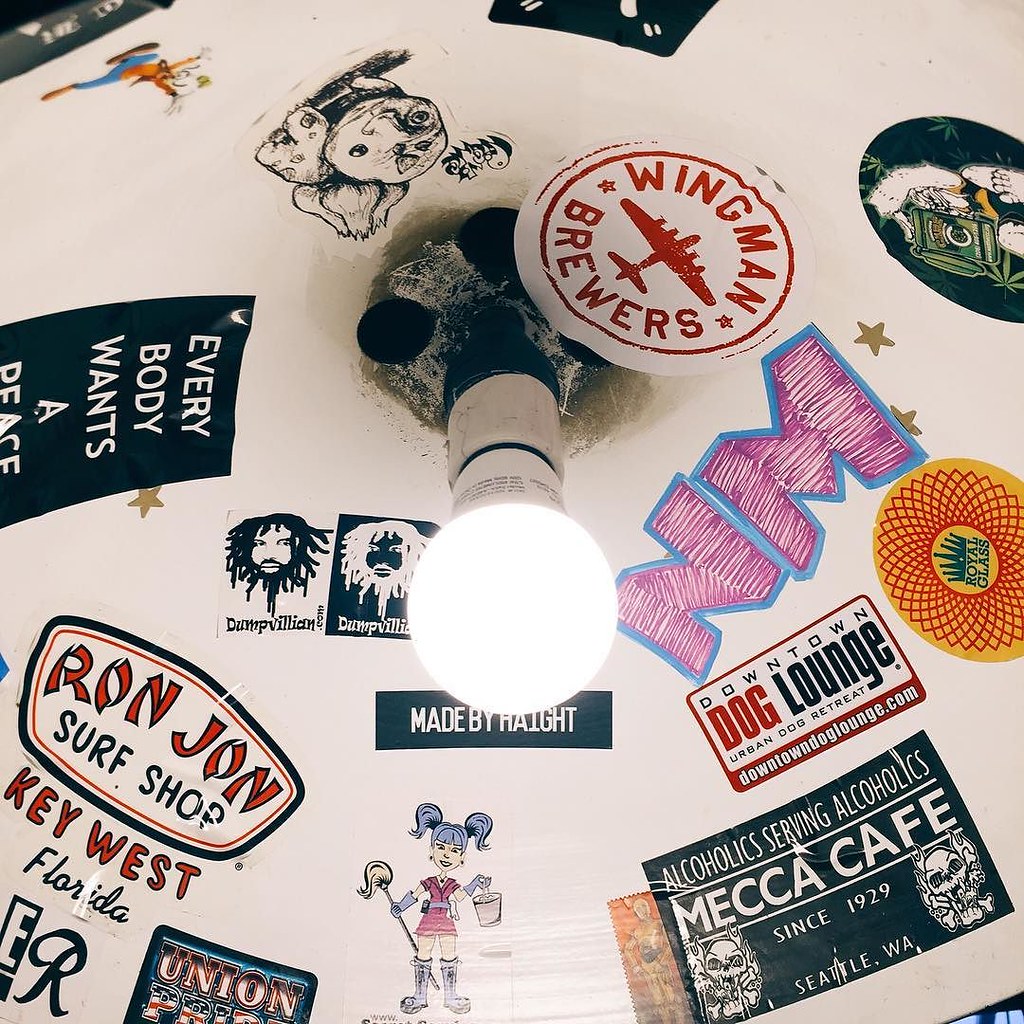The image is a highly detailed color photograph depicting a curved, white ceiling densely covered with various stickers and illustrations. At the center of the ceiling is a bright, round light bulb attached to a short, white column. Surrounding this light fixture are numerous stickers representing different brands and themes. Notable stickers include a red and white circular sticker with a B-52 bomber that reads "Wingman Brewers," a sticker at the bottom left corner reading "Ron Jon Surf Shop Key West Florida," and another at the bottom right reading "Alcoholics Serving Alcoholics Mecca Cafe" since 1929 Seattle Washington, adorned with several skull illustrations. Additionally, to the right of the light are graffiti-style initials "NM," outlined in blue and filled with pink marker, accented with gold stars. The ceiling is a vivid collage of variously themed stickers, some of which are partially cut off or difficult to read, blending elements of photographic representationalism in a chaotic yet visually engaging arrangement.